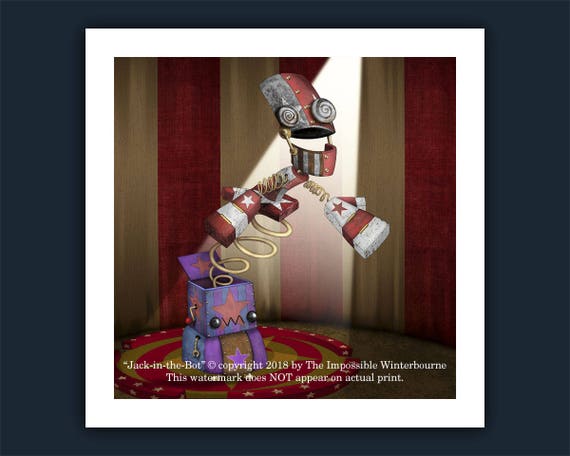This digital illustration features a fantastical, twisted jack-in-the-box set against a black background framed with a white border. Inside this border, the backdrop displays vertical red and white stripes, creating a stage-like setting highlighted by a spotlight from above. The stage itself is brown, centered with a red circular rug adorned with white star markings and concentric rings in red, white, and brown. 

At the center of the rug is the jack-in-the-box. The base of the box is purple with a purple star and is topped by a blue and purple striped square box featuring an orange star on its front. The lid of the box, also blue and purple striped, is open, revealing an orange star on the inside. 

Emerging from the box on a brown, spiral spring is the jack, a peculiarly designed toy with a half-red, half-silver cylindrical head and big, spiral blue eyes. The jack’s face resembles metal with a loosely hinged, semi-circular lower jaw, colored red on our right and divided by white and red stripes with a blue star. Its hands are cement-like and feature a white star on its right and a red star on its left. Both hands and head are connected by gold springs, and the jack appears to be wearing a scarf with alternating patterns of white stars on red and red stars on white, attached to its neck by another spring.

Along the bottom of the image is the caption, “Jack in the Box, Copyright 2018 by The Impossible Winterburn.” Note that the watermark stated in the caption does not appear on actual prints available for order.